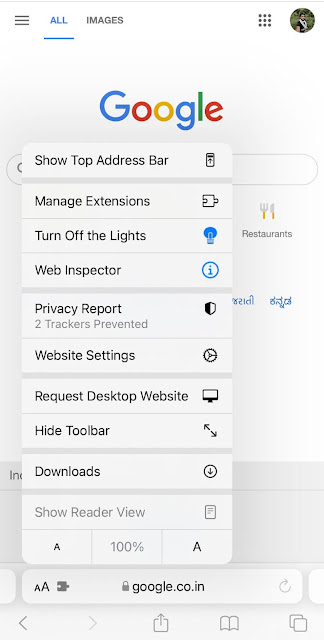The image appears to be a narrow screenshot, likely from a mobile device. At the top, it shows the Google search interface with tabs labeled "All" and "Images", indicated by three horizontal lines. On the right side, there is an icon depicting a person in a suit, and next to it, a square filled with dots. "Google" is prominently displayed in the center of the page in its characteristic colors of red, gold, green, and blue.

A pop-up overlay is visible, displaying a list of options including:
- Top Access Bar
- Manage Extensions
- Turn Off the Lights
- Web Inspector
- Privacy Report
- Website Settings
- Request Desktop Website
- Hide Toolbar
- Downloads
- Show Reader View

Within the pop-up, the screen shows "100%" between two 'A' icons at the bottom.

In the background, partially obscured by the pop-up, is a Google search results page for "restaurants". Some text appears scribbled in blue on the right. The URL "google.co.in" is visible in the search bar at the bottom, along with two 'A' icons to the left. Below the search bar, there are several phone-related images.

This comprehensive description captures the essence and details of the screenshot, providing a clear visual depiction of the various elements present.